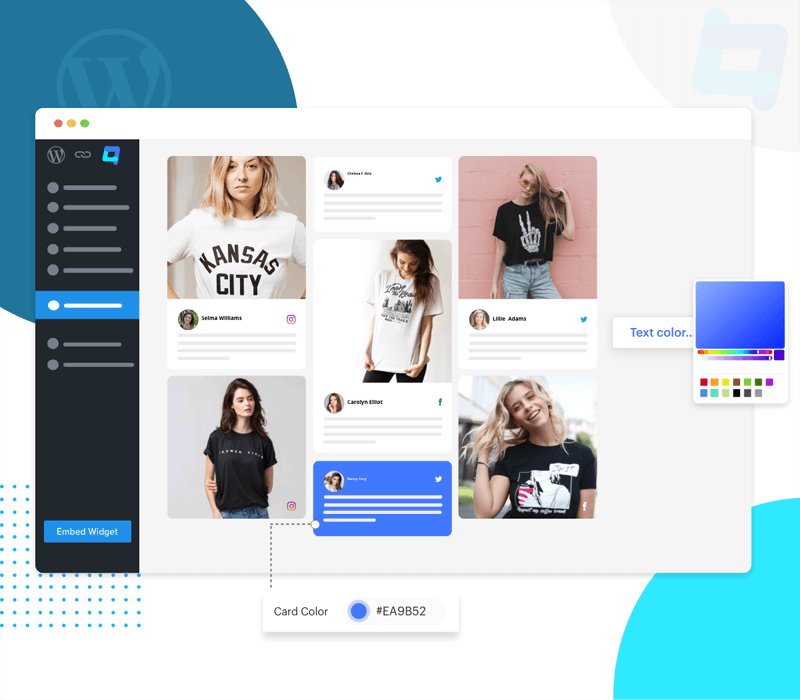The image captures a screen from a shopping website showcasing five different designs of t-shirts worn by young girls. The screen is set against a vibrant background primarily composed of white, featuring circular designs in varying shades of blue. In the lower left corner, a blue grid with dotted lines forms a square against the white backdrop, overlayed by the main image.

The highlighted screen itself has a distinctive black vertical bar on the left side. The upper left corner of the screen includes three small circles colored red, yellow, and green, reminiscent of typical window control buttons.

In the first picture on the upper left, a young blonde girl is seen wearing a white t-shirt with the words "Kansas City" written in black across the front.